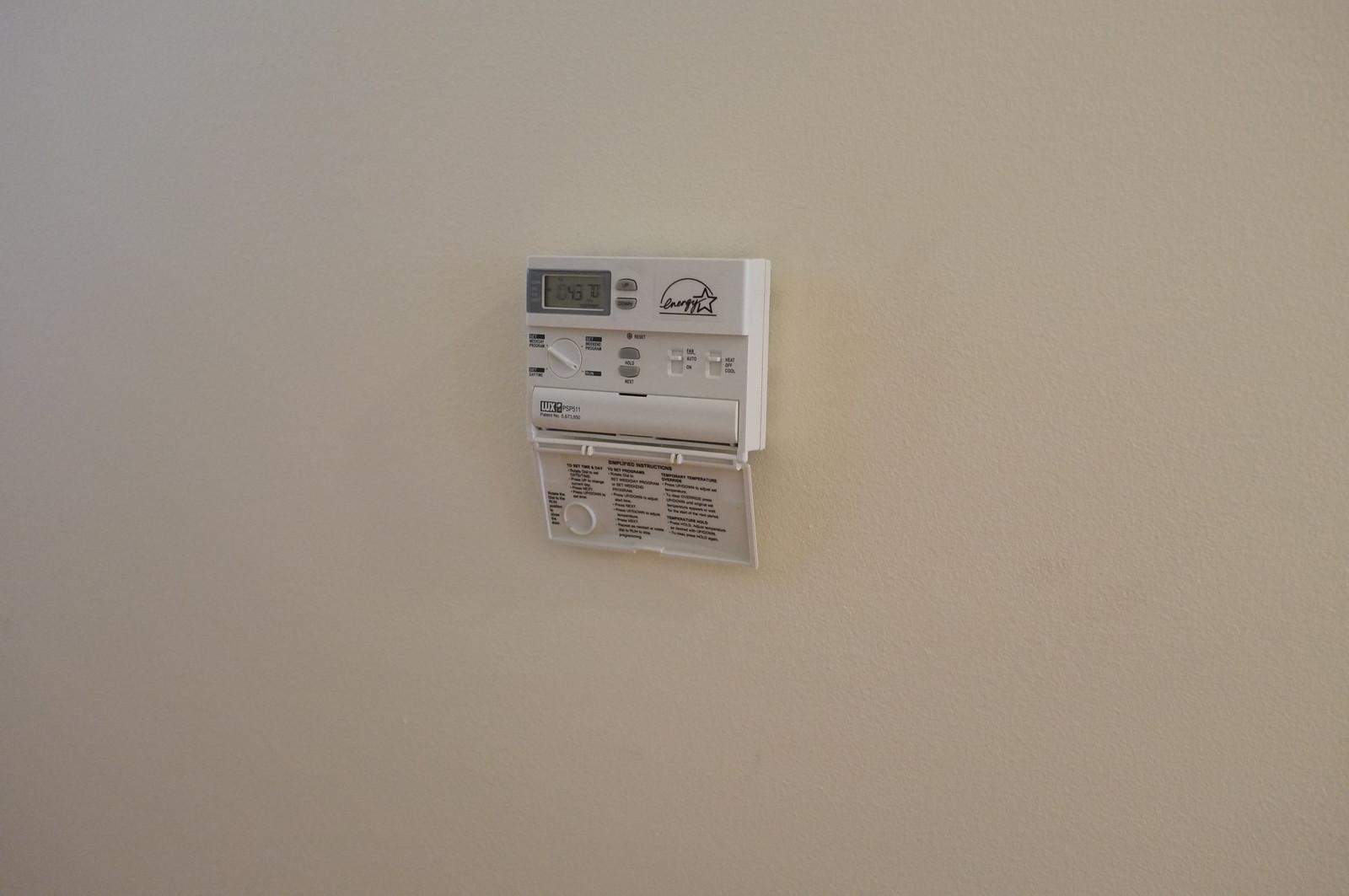The image depicts a meter, likely an electric or gas meter, mounted on a plain white or cream-painted wall. At the center of the image is a small meter box, with its protective flap lowered to reveal the dials and knobs inside. The rectangular meter box is branded "Energy" with a star symbol next to it, located on the top right corner of the box. On the top left, there is a digital screen accompanied by a couple of buttons. Though the numbers on the screen are unclear, they presumably display important metering data. In the middle section of the box, there is a twist dial that can be set to one of four different options. Adjacent to the dial are a few push buttons, while to the far right are two small sliding switches. The bottom third of the box features a cover, likely concealing additional components. Below this cover, the flap is visible, turned upside-down, bearing "Simplified Instructions" at its top, followed by detailed text explaining how to operate the meter.